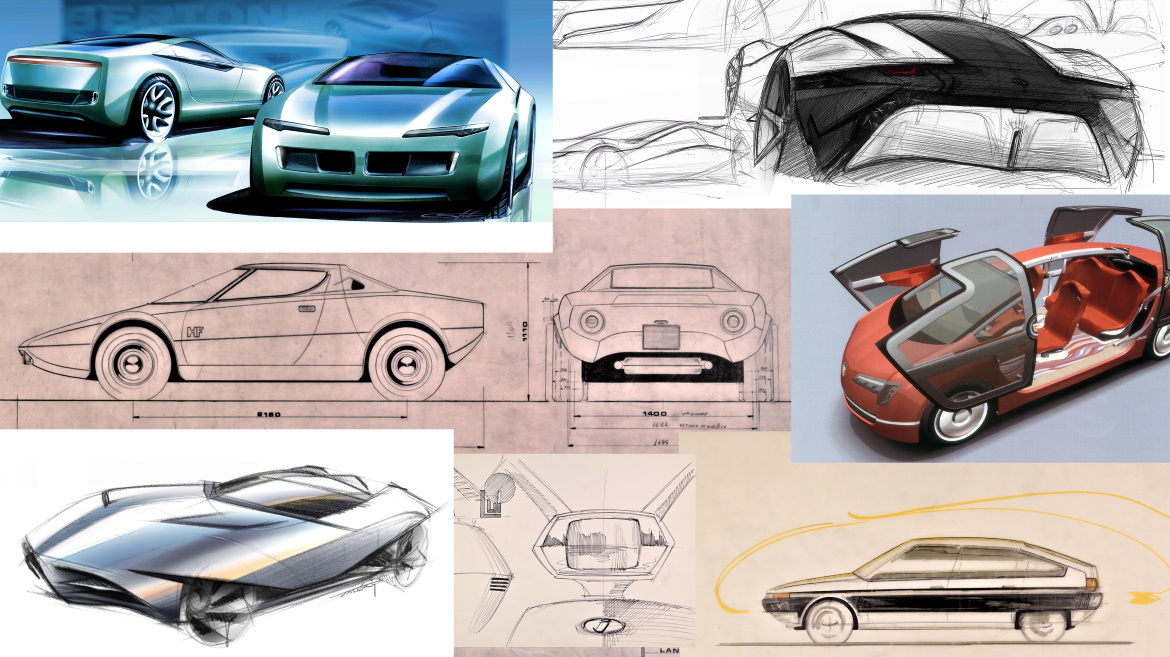This image showcases a series of conceptual car illustrations. There are eight distinct images, combining vibrant full-color depictions and minimalist black-and-white line drawings.

In the top left-hand corner, we see a detailed illustration in shades of blue, green, and white, presenting both the front and back views of a streamlined sports car. The top right-hand corner features a black-and-white side view drawing of a car, offering a simplistic yet clear representation.

The middle left section shows a side and partial rear profile of a car in black and white, set against a light pink background. Adjacent to this, in the middle right, is a full-color image with a striking red car on a blue background. This car has transparent doors that slide to expose the interior, revealing red seats.

Moving to the bottom left corner, another full-color illustration stands out on a white background, depicting a car with a stripe pattern in white, blue, dark blue, and yellow. The bottom middle features a black-and-white illustration on a tan background, viewed from the outside looking into the dashboard of a car. Finally, the bottom right corner presents a side view of a hatchback car in black and white, highlighted by a yellow line arching over its top.